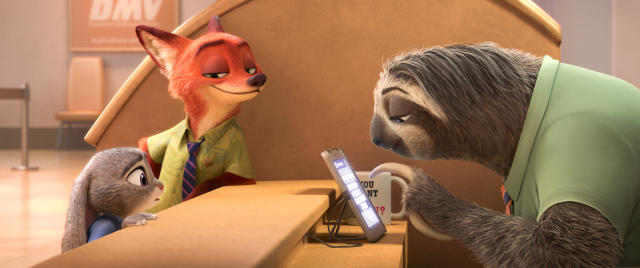The image is a full-color screenshot from the animated movie "Zootopia," set indoors at the Department of Motor Vehicles (DMV). The scene prominently features the DMV sign in red with large white block letters in the upper left-hand corner. At the counter, a humanized fox with a sly smile, dressed in a short-sleeved green button-up shirt and a purple tie, leans casually against the desk. Next to the fox stands a very nervous-looking rabbit child, dressed in blue. On the other side of the counter is a sloth, the DMV employee, who is humorously characterized by his slow movements. The sloth, wearing a green shirt and a tie, is punching on a tablet with one claw while a white coffee mug with black text sits beside the tablet. The scene captures the humor of the notoriously slow service at the DMV through the sloth character's exaggerated sluggishness.